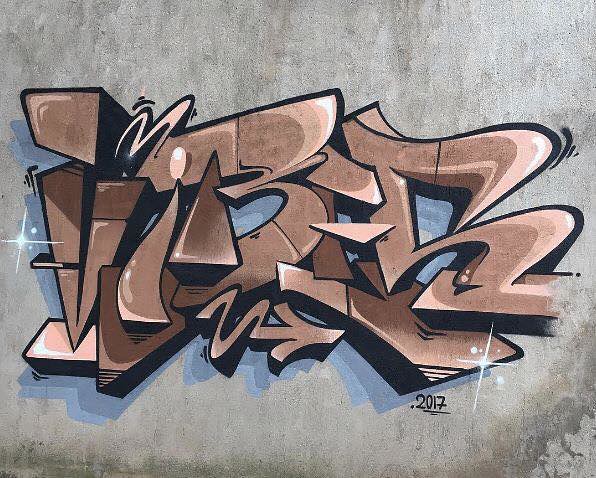A detailed photograph captures an intricately painted graffiti mural on a weathered concrete wall, likely located outdoors near a tunnel or building. The artwork features blocky, three-dimensional stylized text with highly abstract and chunky geometric shapes, including possible letters like V, M, I, B, and R, along with an arrow pointing to the right. Painted primarily in shades of light brown and dull red or peach, the graffiti also incorporates light golden highlights on the upper right-hand edges of the letters, making the design look as if it’s popping off the wall with a sparkling star-shaped flare on the lowest corner. The text casts drop shadows in black and blues for added depth. At the base of the mural, where the concrete appears stained and dirtied with shades of grey, the year "2017" is prominently marked in black. The artwork appears professional, with clever design elements and three-dimensional effects that make the abstract shapes stand out against the rough-textured, unclean surface of the wall.